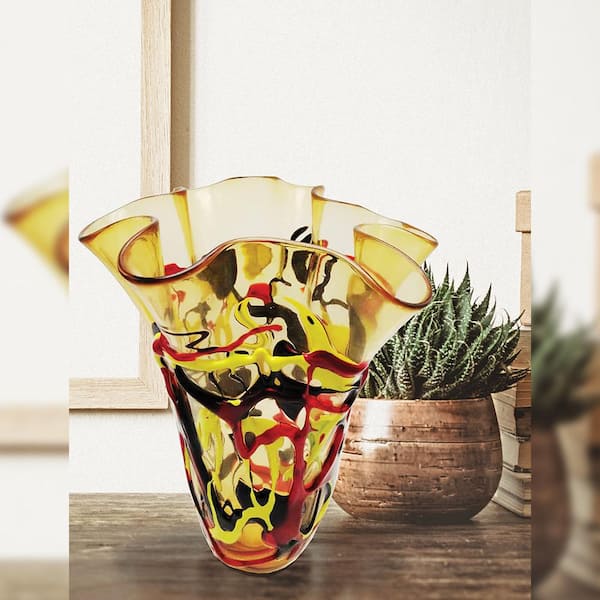The photograph showcases a bright, well-lit indoor scene featuring a multicolored glass vase and a potted plant, both positioned on a wooden table. The vase, ornamented in red, yellow, and black, has a translucent quality and a unique, abstract form resembling folded paper. Its design suggests a bended flower petal shape at the top, seamlessly flowing into a rounded base that rests securely on the table. Beside it, the brown wooden pot houses a healthy green succulent plant with a slightly hairy and fuzzy texture. In the background, the room's natural wood framing and large, bright windows enhance the aesthetic appeal, casting a brilliant white light that illuminates the entire setting.